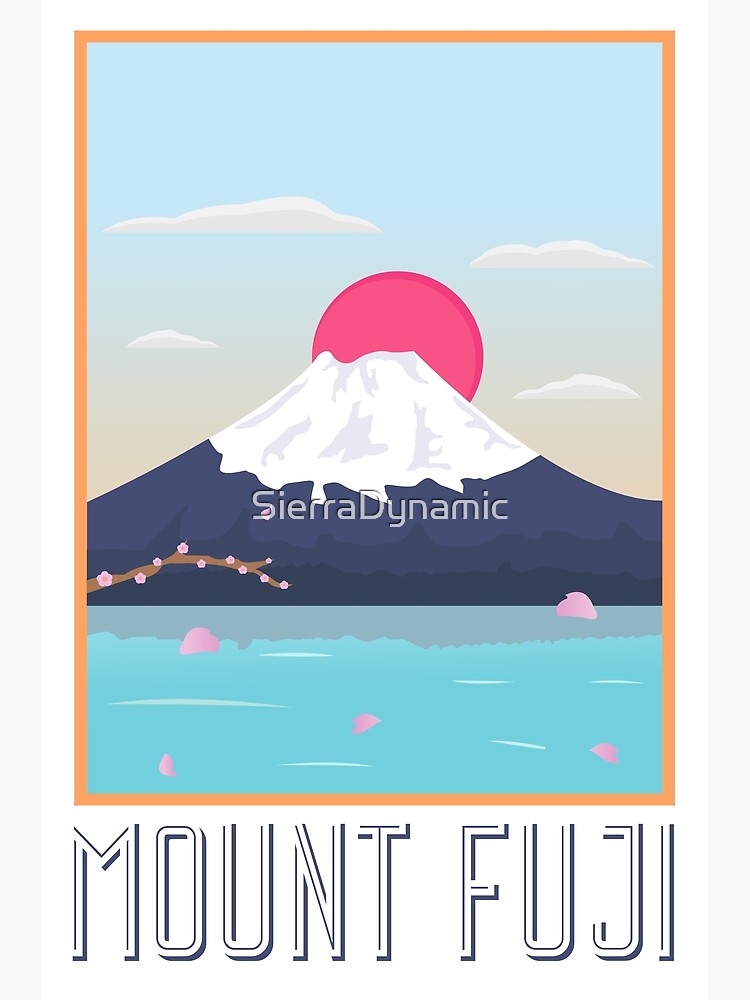This is a detailed and artistically designed poster of Mount Fuji, rendered in simplified graphics. The image is centered around a rectangular frame with notably longer left and right sides. The outermost parts of the left and right margins feature thin gray borders, while the main poster is encased in a white border thicker at the bottom to accommodate blue text reading "Mount Fuji." Beyond the white border is a smaller orange/peach border framing the central illustration.

The main illustration showcases Mount Fuji, depicted with a white snow-capped peak and black lower slopes. Behind the mountain, a large red circle represents the sun, while the gradation of the sky transitions from blue to yellow as it nears the mountain. Below the mountain, a large blue lake reflects part of the peak. The sky is adorned with four fluffy white clouds for added depth.

In the foreground, sakura petals gracefully float through the air alongside a branch laden with pink cherry blossoms. All these elements combined, including the subtle pink hues scattered in the water and across the scene, contribute to a visually appealing and serene representation, likely created digitally. This poster, with its vibrant colors and picturesque design, would make a beautiful addition to any home décor or collection.